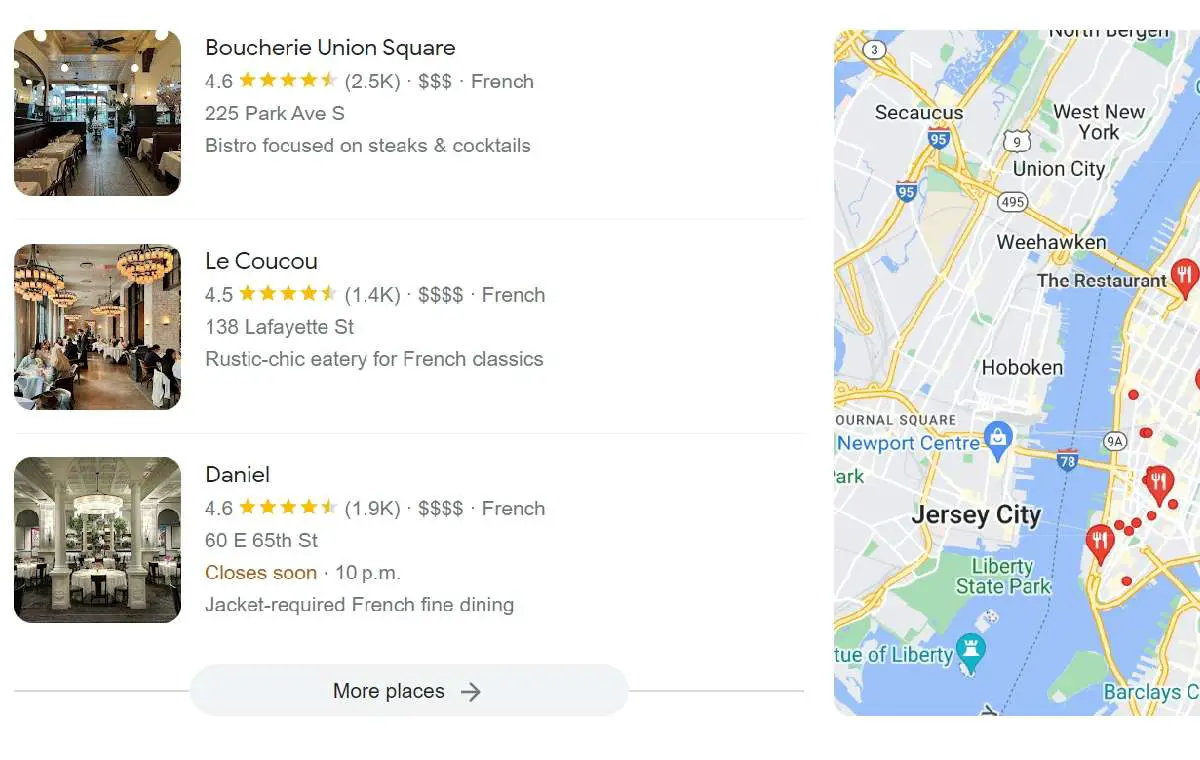The image showcases a search result for French restaurants in the Jersey City neighborhood. On the left side of the screen, there are detailed listings for three French dining establishments, each presented in a vertical arrangement. For each restaurant, there is a thumbnail image followed by the restaurant's name, a star rating, the street address, and a brief description. Below these three listings, there is an option labeled "More places" for additional search results.

On the right side of the screen, a classic Google Maps layout highlights the geographical locations of the three featured French restaurants. Each restaurant's position is marked with a pinpoint on the map, and several additional red dots appear, likely indicating other nearby dining options that aren't included in the primary listing on the left. The overall background of the display is white, providing a clean and clear interface for users.